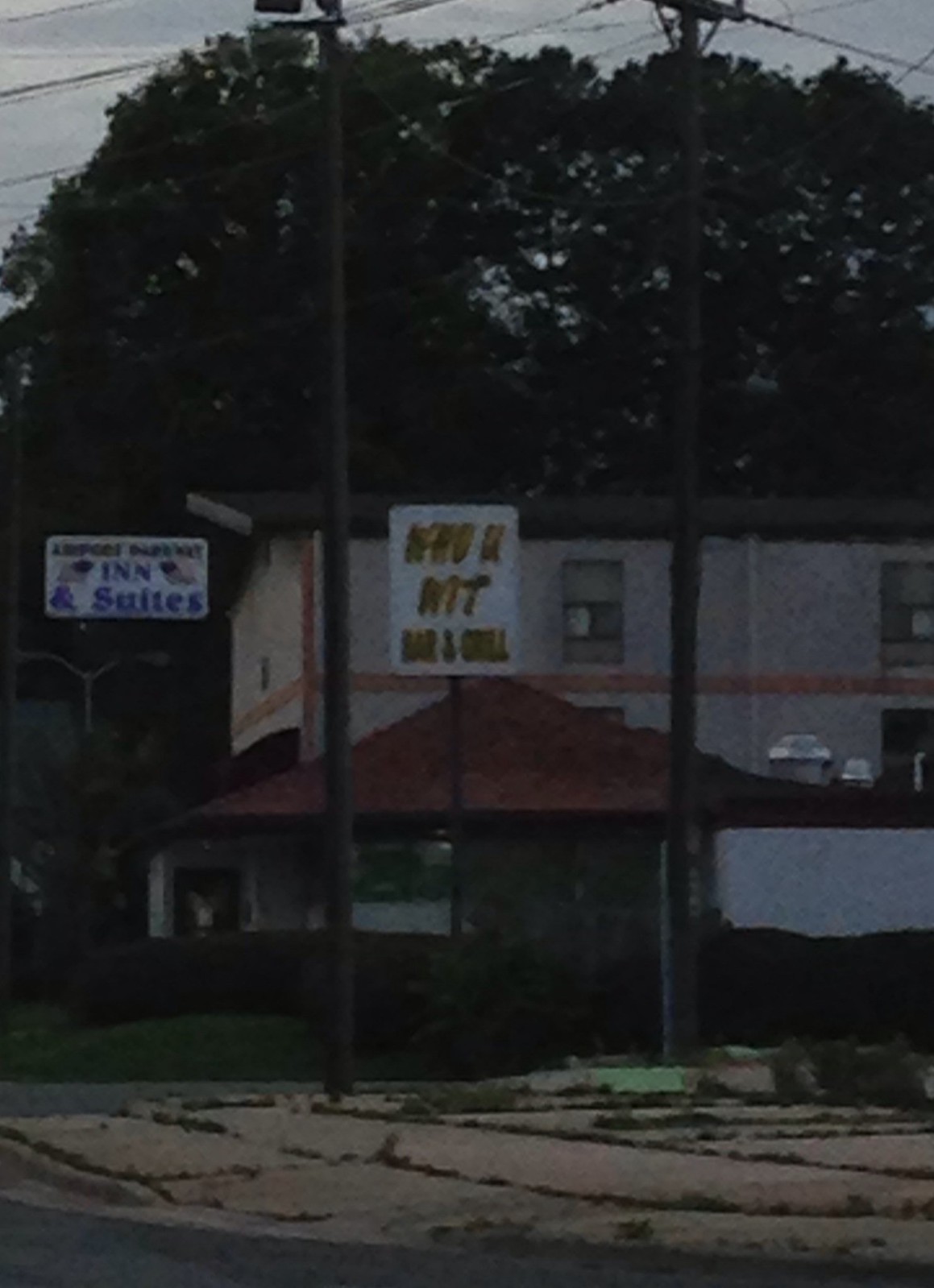In this atmospheric dusk photograph, an exterior view of a light-colored building is captured under the deepening twilight sky. The building prominently features a white rectangular sign hanging out front, emblazoned with the words “Something in Sweets.” A distinctive peach-colored stripe elegantly wraps around the upper middle section of the edifice, delineating the second and third levels. Below this, a prominent reddish-colored triangular roof juts out from the first level, adding character to the structure. In the foreground, the cracked pavement of a nearby lot is visible, with patches of greenery sprouting up through the fissures, hinting at the passage of time. Additionally, two substantial wooden electrical poles rise on the street directly opposite the building, their sturdy forms silhouetted against the dimming sky, completing the textured, moody scene.